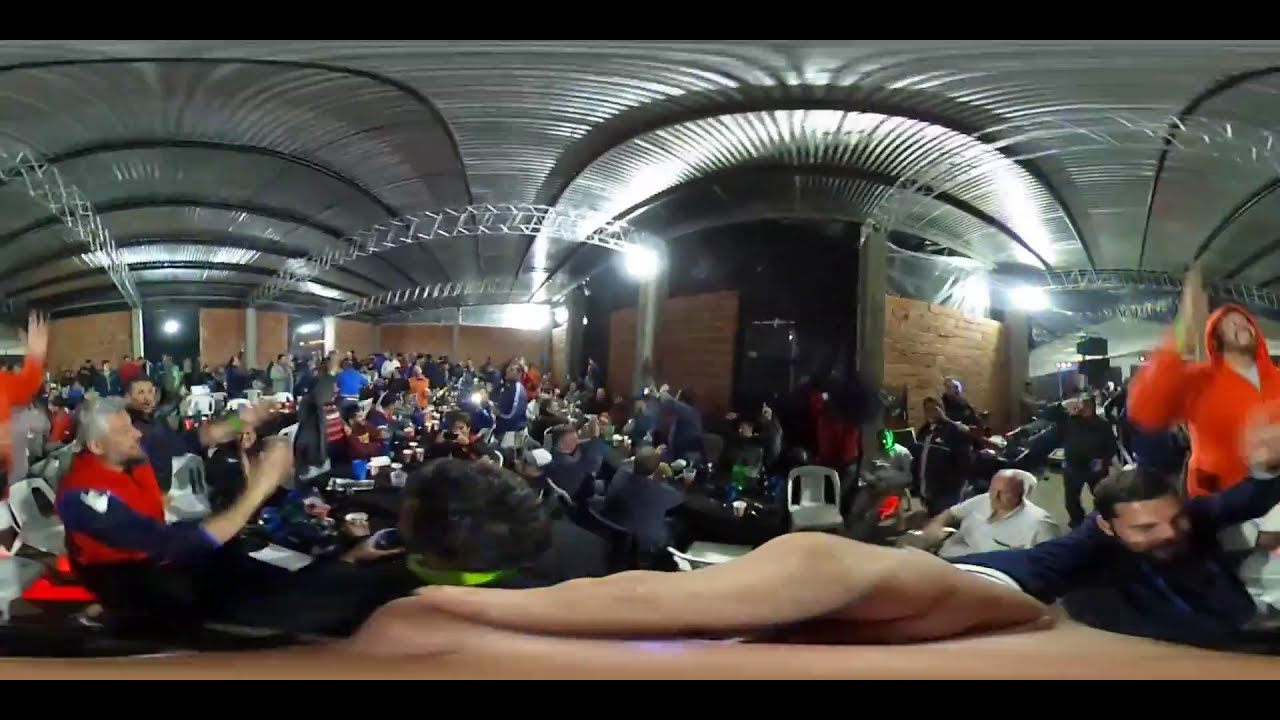The image captures a large, modern hall bustling with a diverse crowd, skewing predominantly male. The room features high, metallic corrugated ceilings and brick walls adorned with decorative, lace-like arches or support beams. The panoramic shot distorts the scene slightly, curving the ceiling and adding a unique perspective. Rows of banquet tables with white plastic chairs are filled with people, many of whom are holding cups. A tan cloth is in the forefront with a man placing his hand on it as if in midst of cheering. It's nighttime, indicated by the artificial lights illuminating the space. The atmosphere is lively with people standing, cheering, and holding up cameras, suggesting a significant event or notable figure at the center of attention, possibly a convention or sports-related gathering. The excitement and energy are palpable, underscored by the collective anticipation and the flurry of camera flashes capturing the moment.